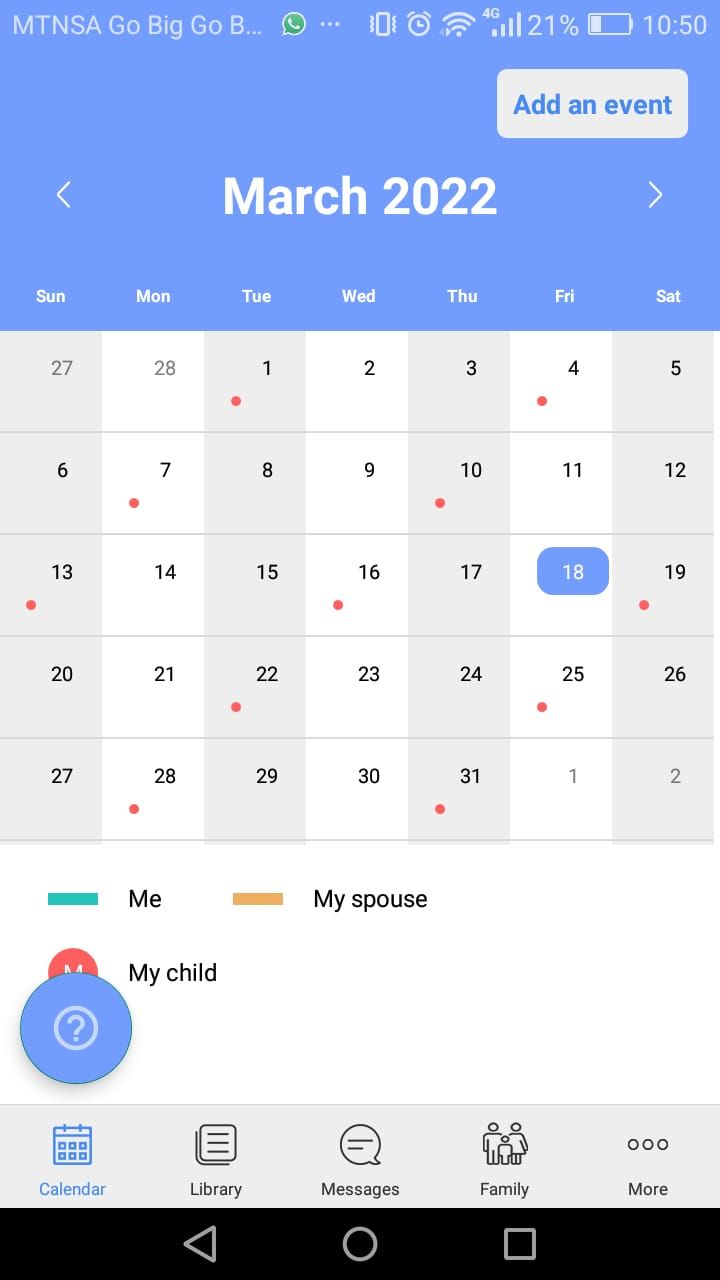This screenshot captures a monthly calendar view on a cell phone, with a clean, predominantly white background. The calendar's interface is rendered in shades of light grey and white, while the header sports a light blue hue. At the very top, typical cell phone indicators are visible against this light blue backdrop. These indicators include the text "MTN SA GO BIG GO B," signifying MTN South Africa as the network carrier. To the right, one can see a phone icon, followed by symbols for Wi-Fi strength, signal strength, and a battery indicator showing 21% remaining. The time displayed is 10:50 AM.

Towards the bottom right corner of the header, there's a white rectangular button labeled "Add an Event" in blue. Centrally positioned within the image, the calendar is set to March 2022, flanked by left and right arrows for navigating between months.

The week commences with Sunday and follows a left-to-right sequence ending with Saturday. The top row features the end of February with the numbers 27 and 28. March starts on a Tuesday (the 1st), with the entire month's days listed accordingly. The bottom row displays the beginning of April, marked by 1 and 2 in a pale font. Various dots are scattered across different dates, signifying scheduled events.

Importantly, the 18th of March is highlighted in blue, indicating the date the screenshot was taken. A key at the bottom specifies the color codes used: green signifies events related to "me," orange represents "my spouse," and red denotes "my child."